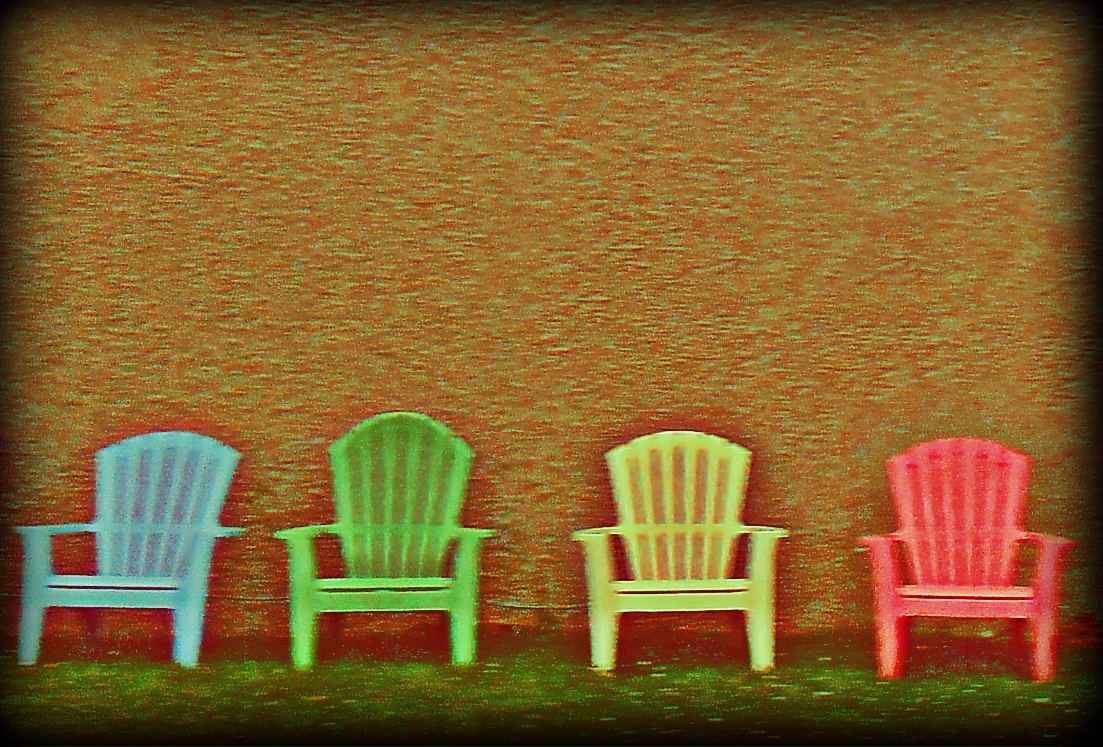The image depicts a slightly blurry, horizontal rectangular illustration that combines elements of a painting and early computer game graphics. The focal point features four evenly spaced Adirondack-style chairs positioned in a straight row on a strip of somewhat unrealistic-looking green grass. The chairs are identical in design, each with vertical wooden slats on the back, and appear to be made of plastic or wood. Their colors, from left to right, are light baby blue, bright lime green, vibrant yellow, and red or dark pink. Each chair casts a subtle shadow behind it, adding depth to the scene.

Behind the chairs is a textured wall, which some observers described as having a tweed-like or mottled appearance, composed of yellow, rust, brown, orange, and occasionally speckled with green and light blue hues. This wall extends down to the grass, merging with the bottom of the image. The outer edges of the illustration are framed with a dark brown or black color, which blurs into the speckled background, giving the overall image a slightly distorted, dreamlike quality.